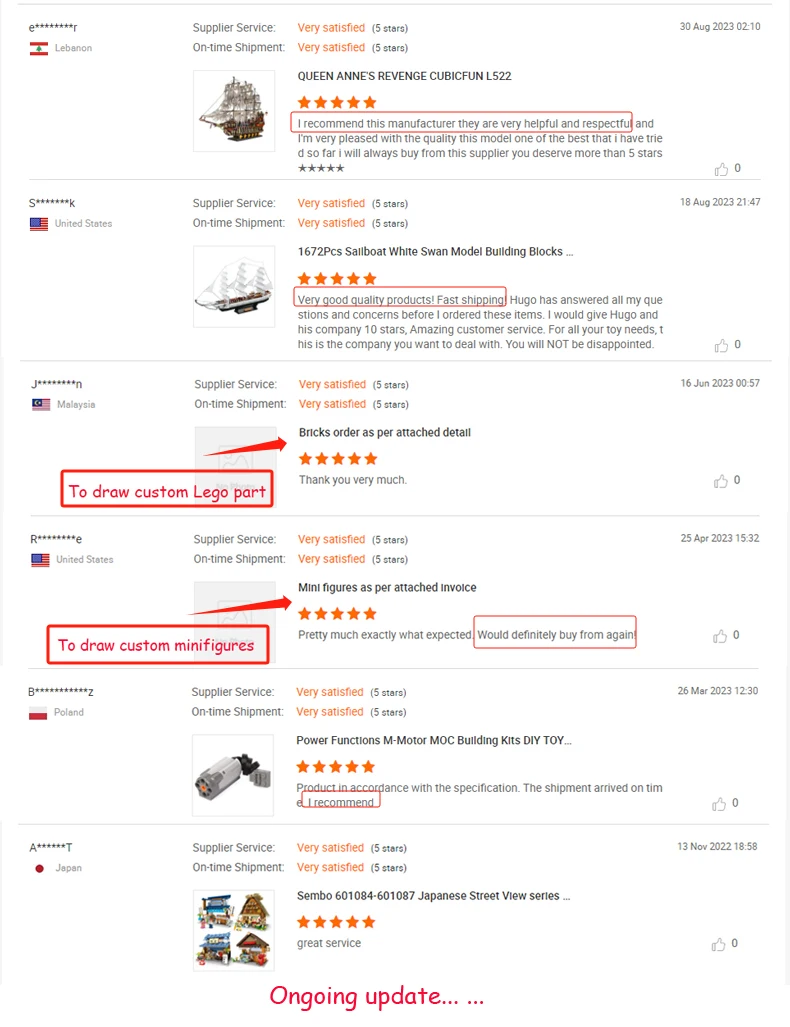This image displays six distinct product reviews, each separated by a thin horizontal gray line. The reviews are organized into three columns: on the left, the review location is noted; in the middle, the supplier service is listed alongside a product image beneath it; and on the right, the name of the product is displayed, accompanied by a rating out of five orange stars, and followed by a short review description. The entire layout is set against a white background, with thin gray lines outlining the left and right sides of the columns. The text throughout the reviews is primarily black with occasional orange text. The image is somewhat zoomed out, making the details difficult to read. At the very bottom, the text "ongoing update..." is prominently displayed in red.